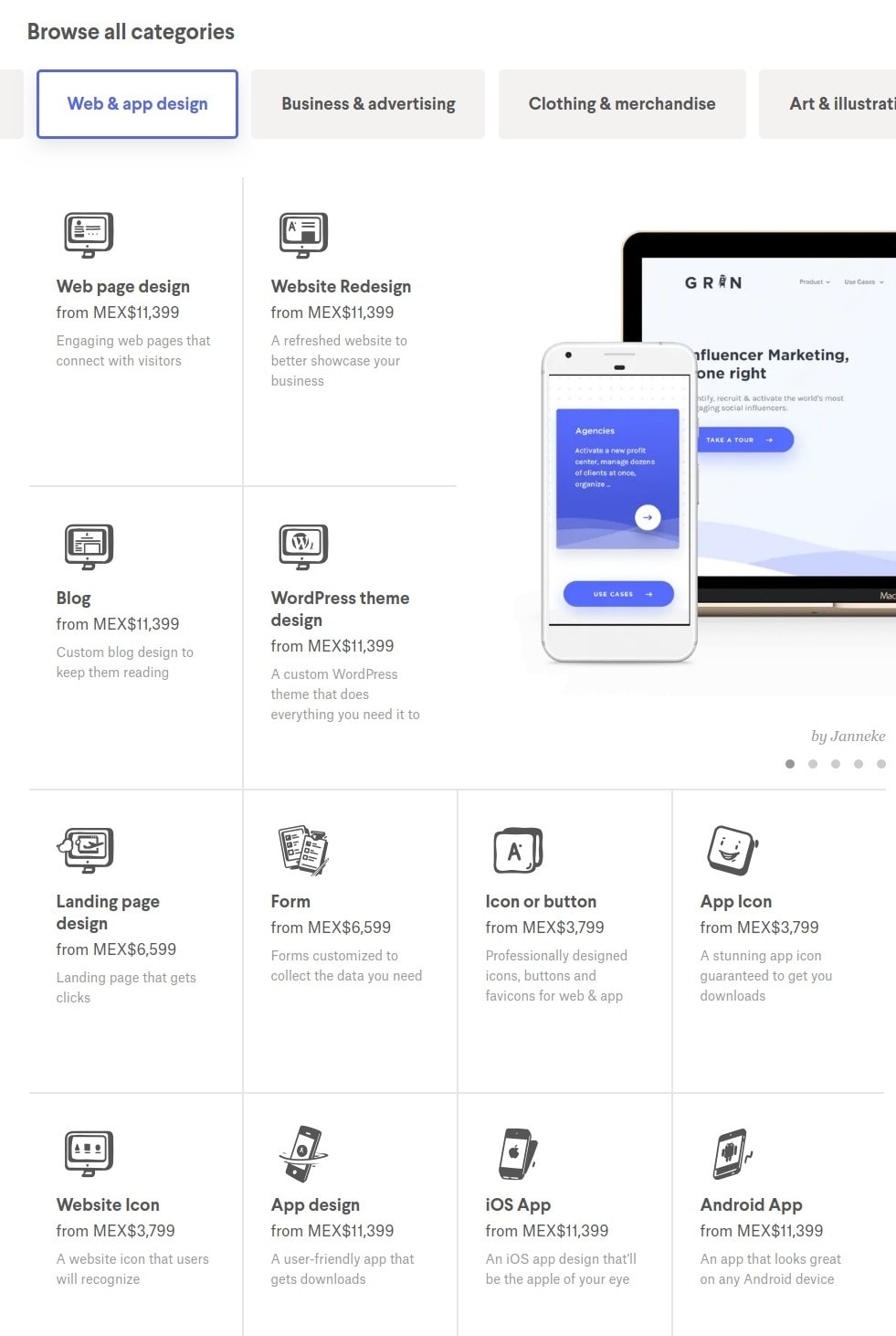This screenshot captures the user interface of a website catering to various digital services. In the foreground, a white smartphone displays a promotional message within a bluish-purple square, which reads: "Agencies, activate a new profit center, manage dozens of clients at once, organize..." A white circle with a purple right-facing arrow is prominently featured at the bottom-right corner of the smartphone screen. Below this promotional message, the text "use cases" can be seen.

In the background, the screen of a laptop is partially visible, partially obscured by the smartphone. On the visible portion of the laptop screen, the text "influencer marketing" appears next to the words "browse all categories" located at the top-left corner. The website is organized with several tabs at the top, with the "web and app design" tab currently selected, highlighted in purple. Other available tabs include "business and advertising," "clothing and merchandise," and "art and illustration."

The content under the "web and app design" category lists various services such as web page design, website redesign, and WordPress theme design, suggesting that users can purchase these digital services. Overall, the screenshot effectively showcases the user interface and navigational elements of a service-oriented website, designed to cater to a variety of professional digital needs.